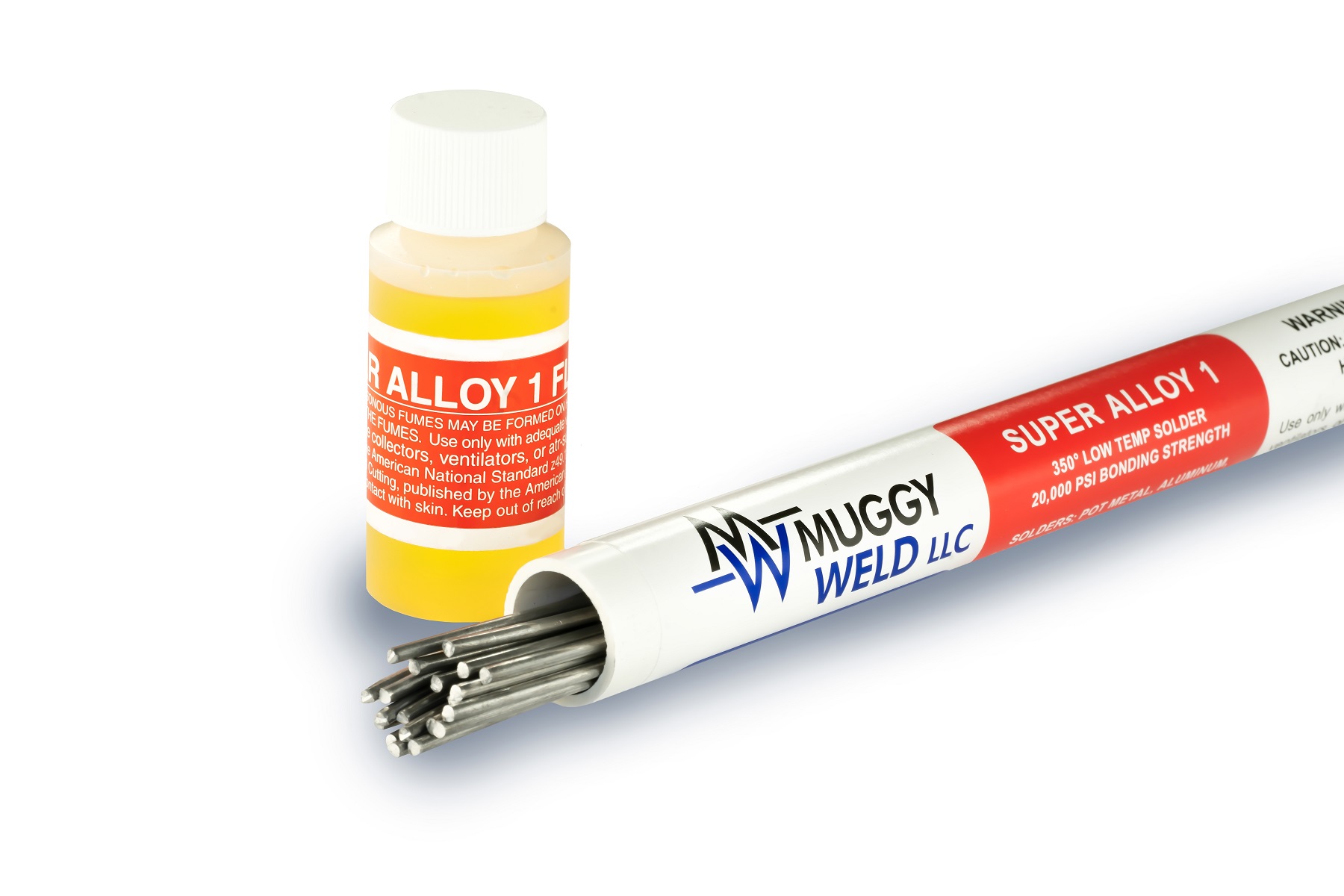In the image, against a stark white backdrop, there are two objects prominently used for alloy purposes. On the left, a clear bottle with a white cap stands upright. The liquid inside is a yellowish-gold color. The front of the bottle features a label with orange and white trimming, displaying “Alloy 1” in large letters. Although much of the text is obscured, visible warnings include phrases like "Flames May Be Formed," "Use Only With Ventilations," and "Keep Out Of Contact With Skin."

Adjacent to the bottle, positioned at an angle, is a white tube containing long, thin metal sticks. The tube primarily exhibits black and blue lettering on the left side that reads "Muggy Weld LLC." In the middle of the tube, a red strip features prominently with white text indicating "Super Alloy 1, 350° Low Temp Solder, 20,000 PSI Bond and Strength." Although the right side of the package is partially cut off, the words “Warning” and “Caution” are discernible.